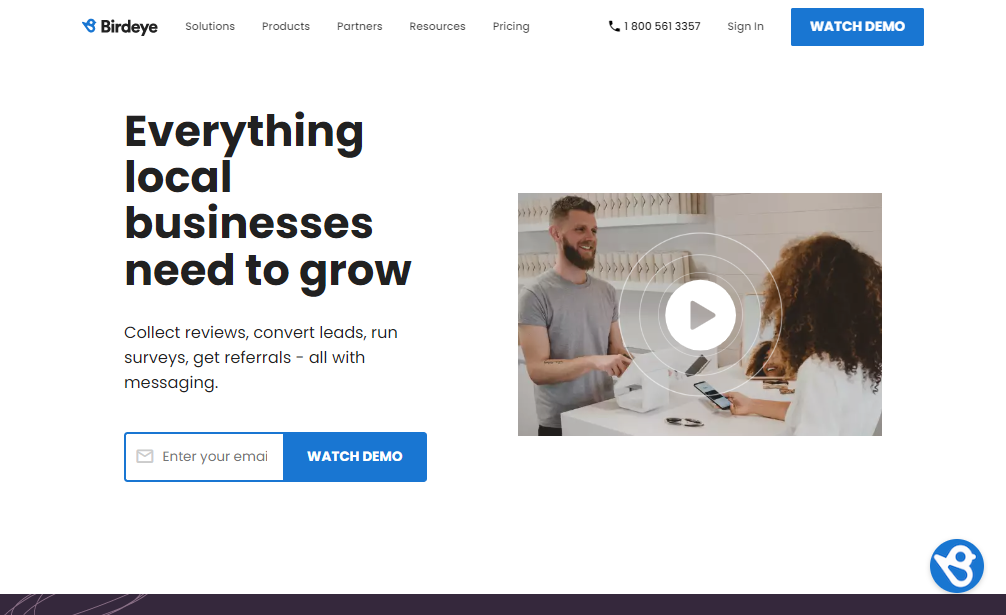At the upper left corner of the image, the BirdEye logo is prominently displayed. To its right, the navigation menu includes sections for Solutions, Products, Partner, Resource, Pricing, and other options such as 1-800-561-3357, Sign In, and Watch Demos. There is a notable blue button with white text that also says "Watch Demos."

The headline, "Everything local businesses need to grow," is the largest text on the page, meant to catch the viewer's attention. Beneath it, a series of actions are listed in smaller font: "Collect reviews, convert leads, run surveys, get referrals, all with messaging."

Further down, there is a call-to-action field where users can enter their email, highlighted by a blue outline on a white background, with the text in gray. Adjacent to this is another blue button with "Watch Demo" written in white.

The right side of the page features an image of a man standing behind a counter and a woman seemingly purchasing something from him. A white play button with a gray arrow overlay suggests that this image is clickable for a video or demonstration.

A thick black line signifies the bottom boundary of the website. The entire layout is set against a white background, with a color scheme incorporating gray, black, white, blue, and natural tones from the photograph of the people. The woman's hair displays hues of brown, black, and orange, adding a touch of vibrancy to the otherwise minimalistic design.